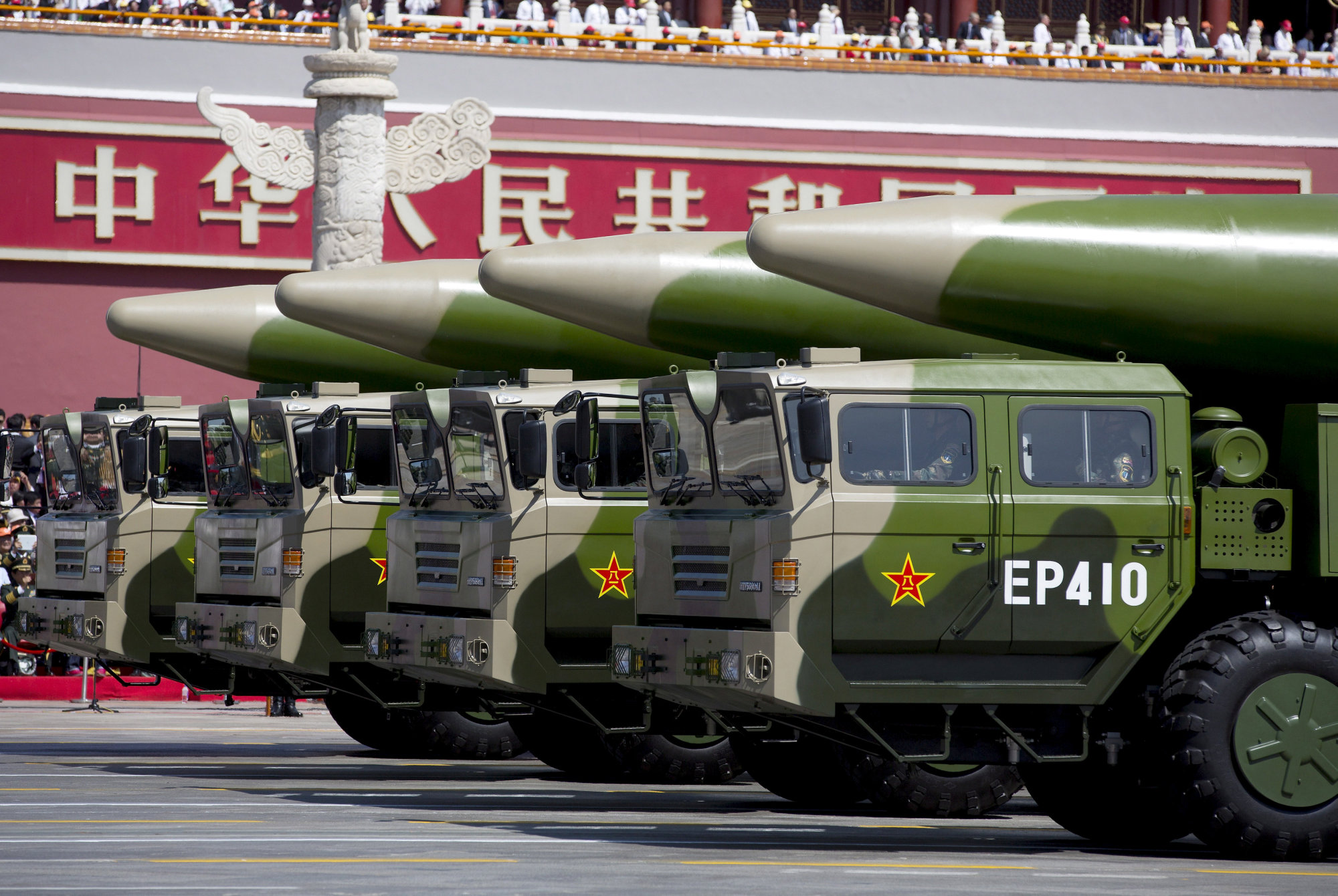The image depicts an outdoor military parade, likely taking place in China or North Korea, under the bright Sun. Four large, green camouflage tanks are lined up side by side on a concrete road with yellow lines. Each tank features prominent yellow and red stars on the doors and displays the identifier "EP 410." The tanks are equipped with silver grills, front hitches, and possess both side and front windows. Mounted on top of the tanks are green and white missiles. Above the tanks, a red banner adorned with white Chinese lettering is visible. Bordering the scene is a gold railing, behind which a crowd of spectators stand and sit, observing the parade. The overall scene conveys a sense of military readiness and is marked by the presence of large, imposing vehicles.